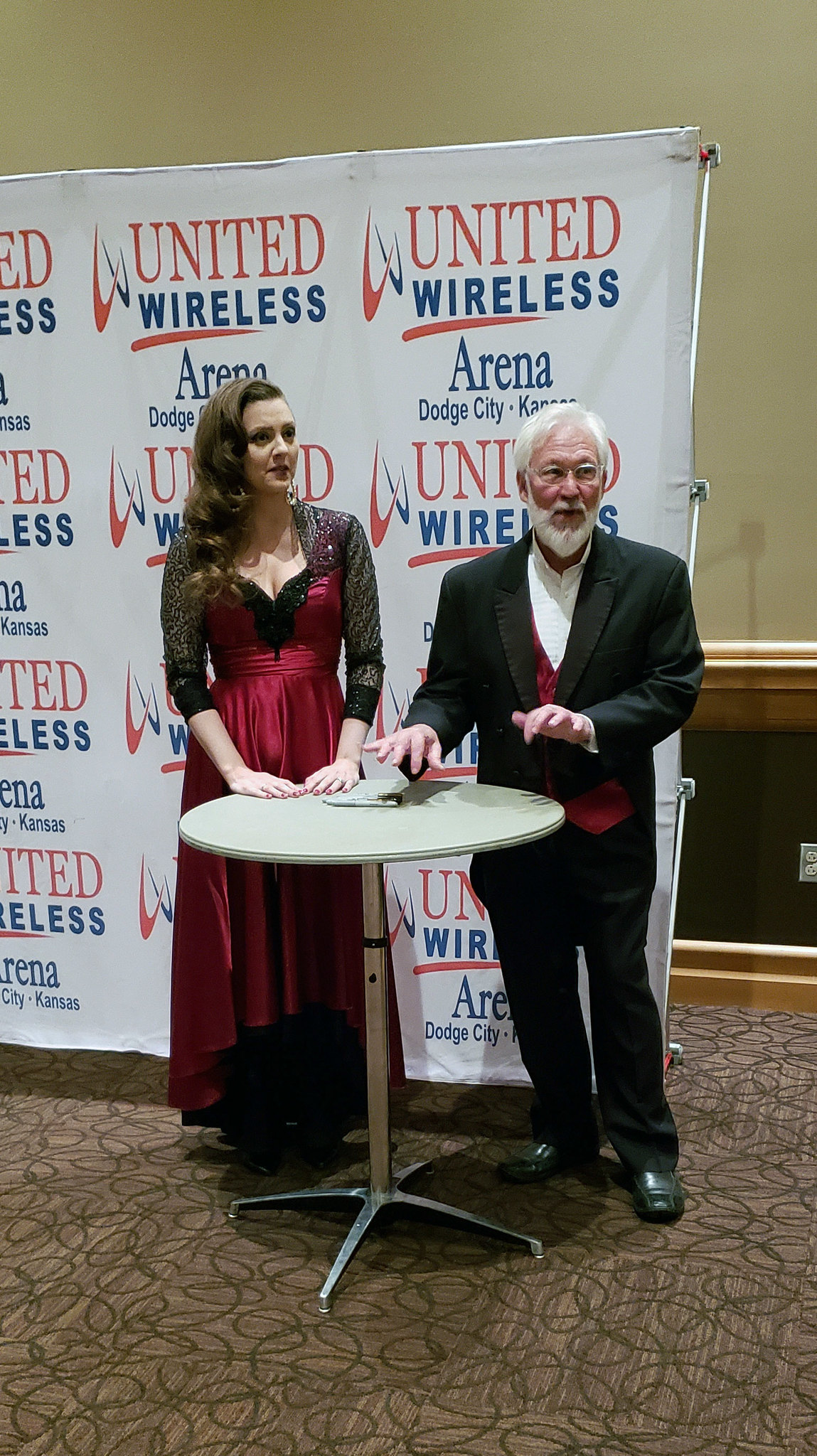In this indoor conference setting, a distinguished older man with white hair, a matching beard and mustache, stands beside a woman at a small, tall round table with silver legs. The man is dressed in a dark suit adorned with red accents, a shiny burgundy vest, and a high-collared, white shirt; he’s seen pointing downwards with one hand and holding papers with the other. Beside him stands a younger woman in an elegant, long red evening gown, which features a black lace bodice and long sleeves. Her brown, curly hair cascades over her left shoulder. They are positioned in front of a large, white backdrop that repeatedly reads "United Wireless Arena, Dodge City, Kansas" in bold red and blue letters. The backdrop covers a beige wall with dark paneling at the bottom, and the floor beneath them is a textured, swirly patterned carpet.